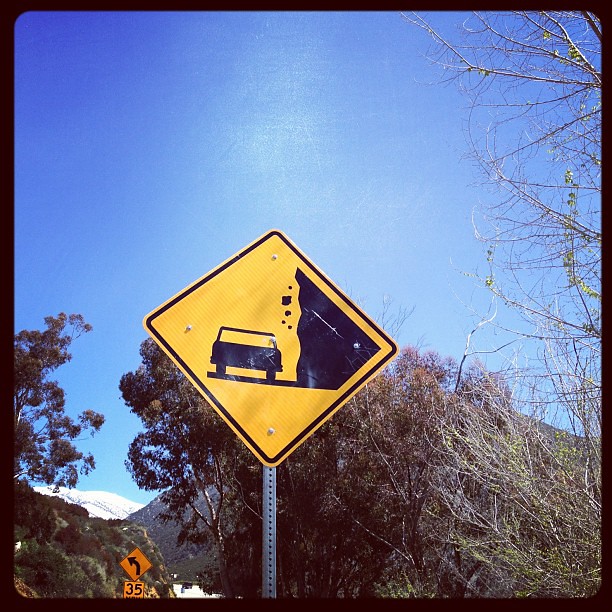A crisp photograph captures a scene framed in a thin black trim, presenting a vertical vantage point that is both dynamic and detailed. Central to the image is a prominent yellow diamond warning sign, cautioning drivers of potential falling rocks from an adjacent cliffside. The vivid yellow sign, featuring a graphic representation of a car and tumbling rocks, is set against a backdrop of a serene, clear blue sky that occupies the upper half of the image.

The background is enriched with the tops of slender-branched trees sparsely adorned with leaves, adding texture and depth. Dominating the bottom third of the image is a distant, tree-covered mountain, partially veiled by the thin trees in the foreground. To the left, beyond this forested peak, another mountain emerges, its snowy white cap hinting at a higher elevation.

Near the bottom left corner, a small portion of the image (less than 5%) reveals a secondary yellow diamond sign indicating a sharp turn ahead with a speed limit of 35 miles per hour. Below this sign, a glimpse of a grassy cliff is visible, with more trees perched above it, blending seamlessly into the scene. The harmonious balance of natural elements and clear signage provides a picturesque yet cautionary view, encapsulating the beauty and inherent risks of this mountainous landscape.